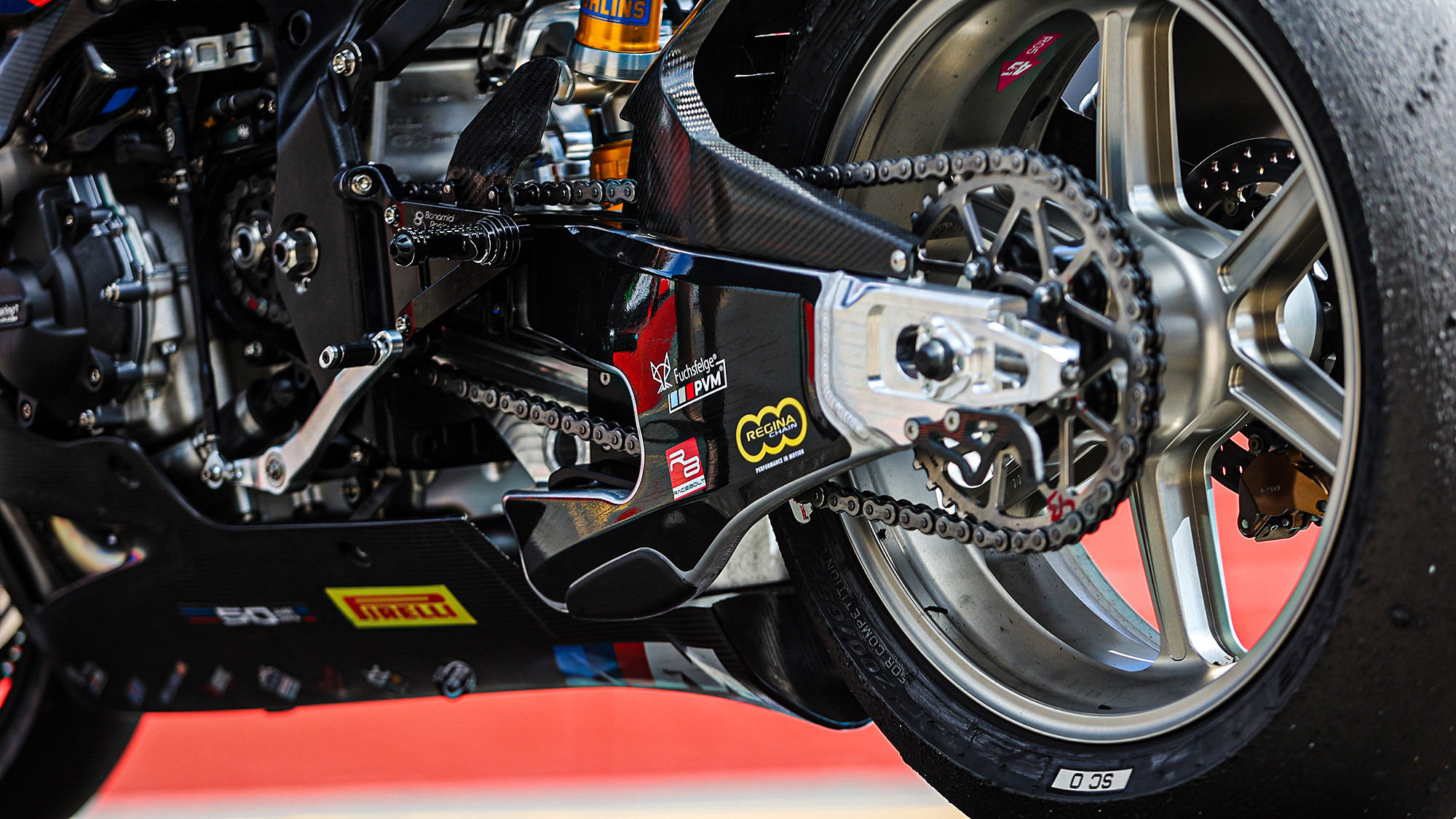The image showcases a close-up of a motorcycle wheel, emphasizing its technical and stylized elements commonly seen in automotive magazines. The horizontal photograph highlights the intricacies of the motorcycle's rear wheel assembly. Prominent features include the silver rim and metal components, contrasted by various black parts. The chain, emblazoned with "Regina Chain" within three yellow circles, wraps around the wheel, which also displays a Pirelli sticker. Further details include the designation "SC0" in a small rectangle at the bottom of the wheel. The motorcycle’s tire is partially visible, adding depth with hints of blue and red accents, capturing the essence of high-performance engineering.